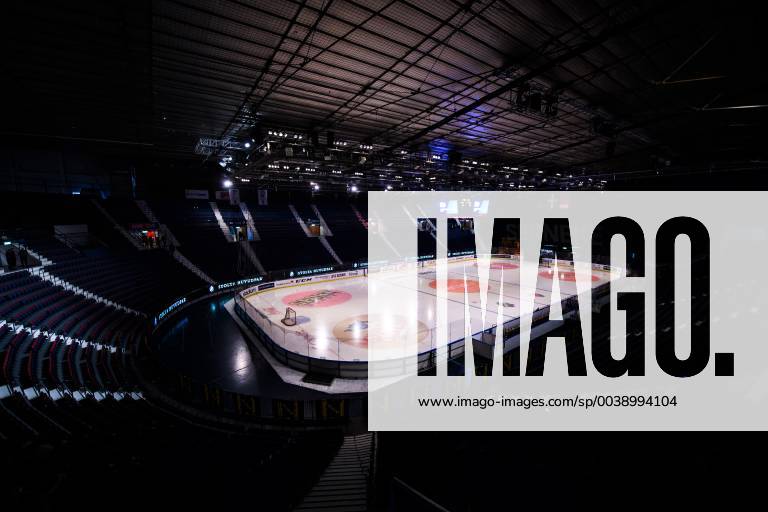The image is a dark, atmospheric photograph of the interior of an empty hockey arena, likely being used as an advertisement for a photography or digital image service. The arena is mostly unlit, except for some lighting between the aisles of the stands and the well-lit white ice floor, complete with a goalie net on the left-hand side. Dominating the foreground is a large cream-colored rectangle extending from the right into the center, featuring the translucent black letters "IMAGO" through which the ice rink is visible. Beneath the logo is a black square, followed by the text www.imago-images.com, "SP", and "003-899-4104." The image appears both on their website and suggests contact details, indicating this might be a purchasable print from Imago's catalog.